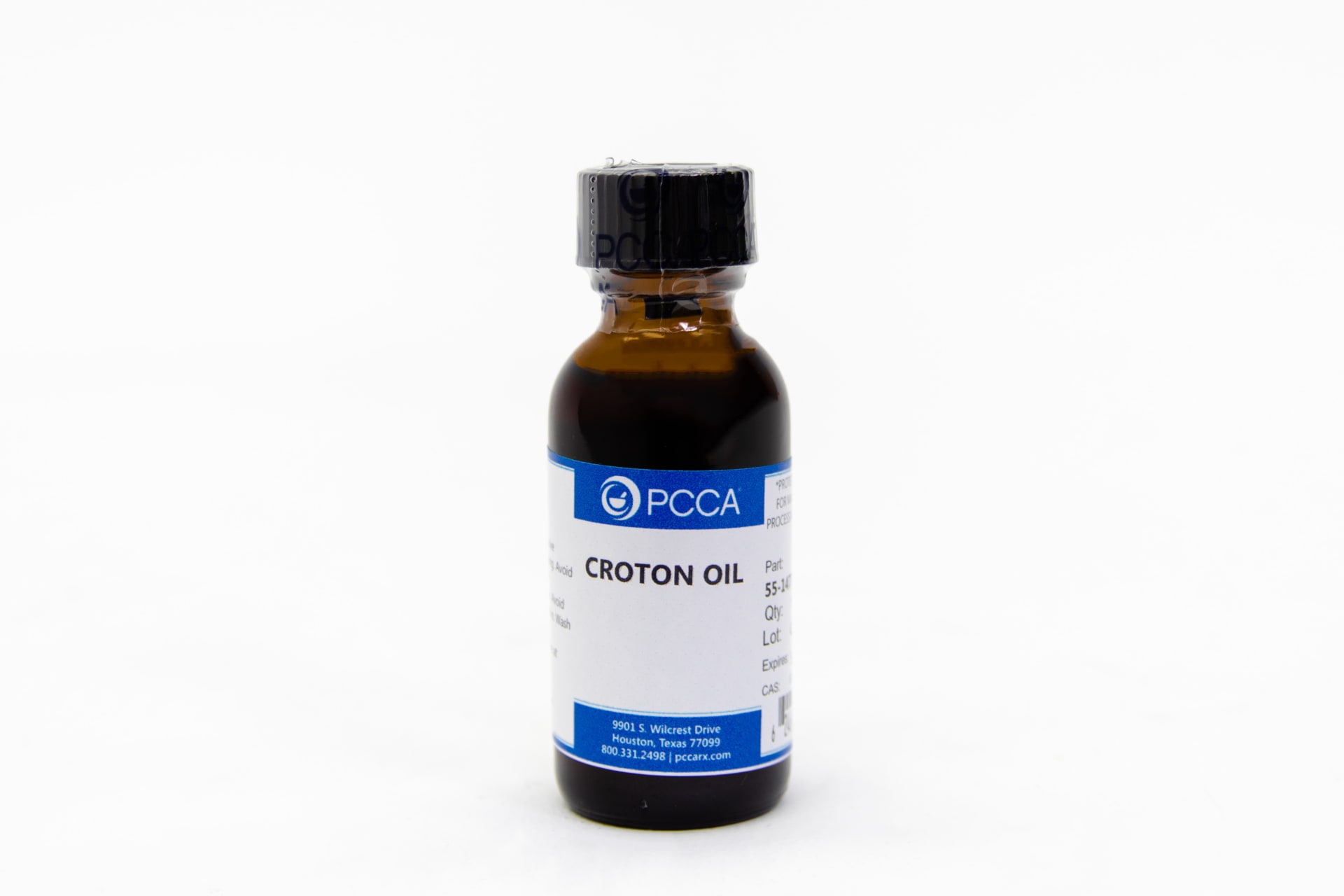The image features a small medical bottle, approximately two to three inches tall, made of brownish glass with a black cap. The bottle is wrapped in a clear plastic seal, with a perforation for easy removal. The label on the bottle is primarily blue and white. A blue bar at the top contains the text "PCCA" in white alongside a logo. The center of the label is white with bold black text reading "Croton Oil," and additional black text providing details, though somewhat distorted due to the bottle's curvature. At the bottom of the label, another blue bar includes white text with the address "9931 South Wilcrest Drive, Houston, Texas 77099" along with a phone number and the URL "PCCARX.com." The bottle appears to be filled with a brownish liquid. The entire setup is displayed against a white background.